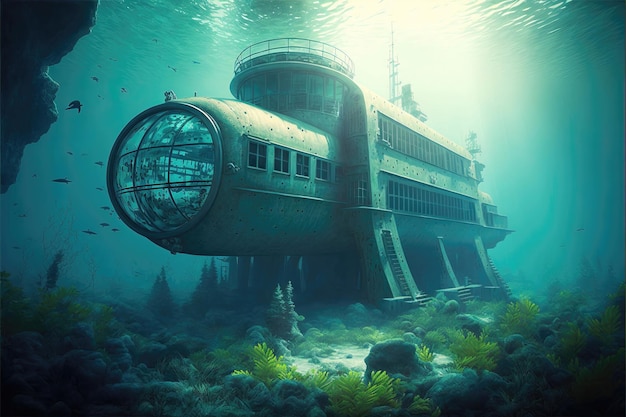The underwater image depicts what appears to be a submerged, fantastical vessel or submarine resting on a teal blue ocean floor. The foreground is dominated by a striking glass dome at the front of the vessel, which faces left and is sectioned into nine squares by black lines. This cylindrical front maintains its round shape while extending towards the back, where it transitions into a more squared structure. Windows are aligned along two visible levels, indicating two floors.

At the top of the vessel's cylindrical section, a circular tower rises, encircled by a metal guardrail, and crowned with a very large antenna. Below, substantial metal legs anchor the vessel to the seabed, with steps visible on the front and back legs, all colored green with white highlights. The surrounding water is illuminated by light beams piercing through, casting waves and reflections around the vessel. The seafloor features scattered green plant life and a mix of white sand. A notable black rock formation occupies the upper left corner, and the lower right corner is filled with fuzzy-looking green vegetation. Numerous fish and other aquatic creatures swim around the submerged vessel, contributing to the vibrant underwater scene.